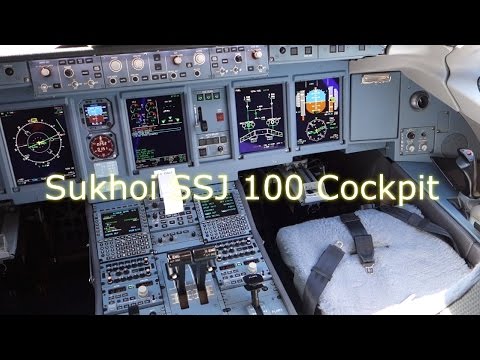The image is a detailed video still showcasing the cockpit interior of a Sukhoi SSJ-100 airplane. The top and bottom of the image are framed with thick black borders indicative of a video still. Prominently written in white text across the center of the image is "Sukhoi SSJ-100 cockpit." 

To the left, there is a white pilot seat with black seat belts draped across it. The cockpit itself is gray and features a complex array of controls. Directly in front of the seat are four large rectangular screens used for vital flight information such as elevation and degrees, flanked by two smaller square gauges. 

Above these displays, there is an extensive overhead panel loaded with numerous buttons and knobs, stretching the length of the cockpit. The center console includes three distinct levers and is outfitted with six panels containing a variety of buttons and switches. The intricate arrangement of dials, joysticks, and throttles on the dashboard highlights the advanced technology and design of this aircraft's control system.